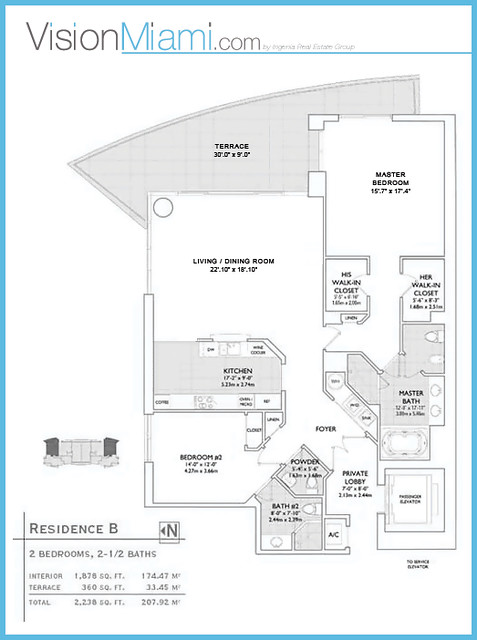Here is a cleaned-up and detailed caption for the described image:

This image appears to be a black and white screenshot from a magazine featuring blueprints, enhanced with subtle blue highlights. The top of the image displays the website "visionmiami.com" with "vision" in black text with blue dotted 'i's, "miami" in blue text with black dotted 'i's, and "dot com" in black text. It includes a small, partially legible note indicating affiliation with a real estate group.

The blueprint depicts a detailed layout of a residence labeled "Residence B." The specifications in the bottom left corner state that it includes two bedrooms and two and a half baths, with an interior area of 1,876 square feet (174.747 square meters) and an additional terrace area measuring 360 square feet (33.45 square meters), making a total area of 2,236 square feet (207.92 square meters). 

Key rooms and features labeled in the blueprint include the terrace, master bedroom, living and dining room, two walk-in closets, master bath, kitchen, second bedroom, private lobby, foyer, powder room, and an additional bath. Although some text and numbers are blurred, the blueprint provides a clear and comprehensive layout of the residence.